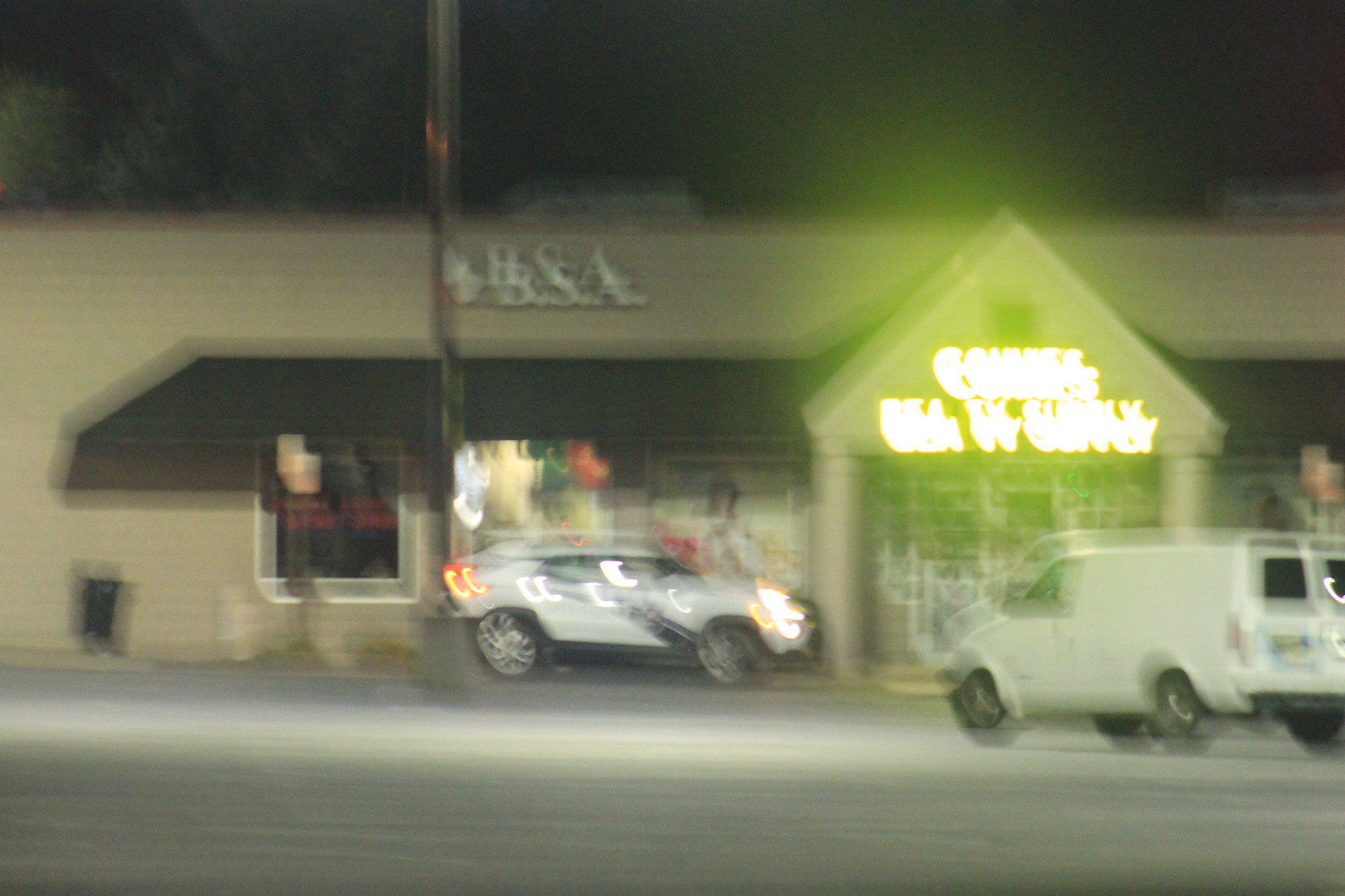This nighttime photograph features a vibrant parking lot in front of a single-level commercial building with a distinctive plaza-style architecture. The image is noticeably blurry, giving a doubled appearance to its elements. At the forefront of the photo, a white van faces the store, while next to it, a white police-style SUV or sport vehicle is parked sideways directly in front of the building. Overhead, the building's facade displays a prominent, though unclear, logo that likely reads "BSA" in white letters. Dominating the entrance is a triangular, well-lit canopy with an almost glowing neon sign whose text remains unreadable due to the blur. Supporting its structure are two pillars, forming a covered walkway leading into the store. Additional light sources, including street lamps and the intense reflections from the neon sign, illuminate the area, casting a vibrant glow over the parked vehicles. A telephone pole is also visible to the left of the white vehicle, blending into the illuminated yet indistinct storefront, which is partially obscured by paper adverts in the windows.